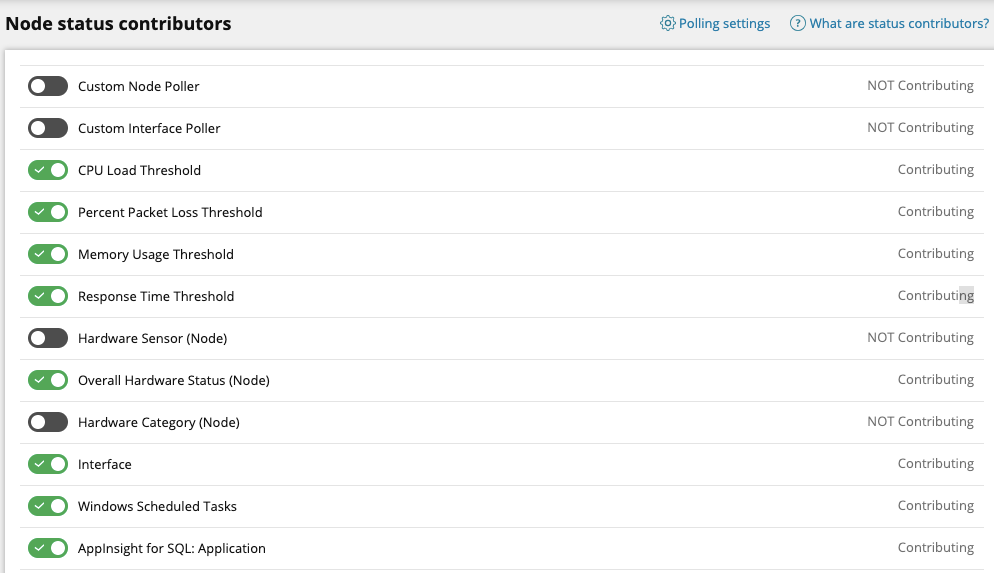This image is a detailed screenshot of a user interface dedicated to node status contributors. Located in the upper left-hand corner, the title "Node Status Contributors" is clearly displayed, while the upper right-hand corner features two sections labeled "Polling Settings" and "What Are Status Contributors?".

Running vertically down the left side of the interface are a series of toggle switches. The initial two switches, labeled "Custom Node Poller" and "Custom Interface Poller," are turned off. Following these, the next four switches are activated and labeled respectively as "CPU Load Threshold," "Percent Packet Loss Threshold," "Memory Usage Threshold," and "Response Time Threshold."

Subsequently, another toggle button is turned off, labeled "Hardware Sensor Node." The next switch, labeled "Overall Hardware Status Node," is enabled, whereas the following switch, named "Hardware Category Node," is turned off. The remaining three switches are all turned on and are listed as "Interface," "Windows Scheduled Task," and "AppInsight for SQL Application."

This organized layout allows for quick identification and status checking of various network and hardware monitoring elements.